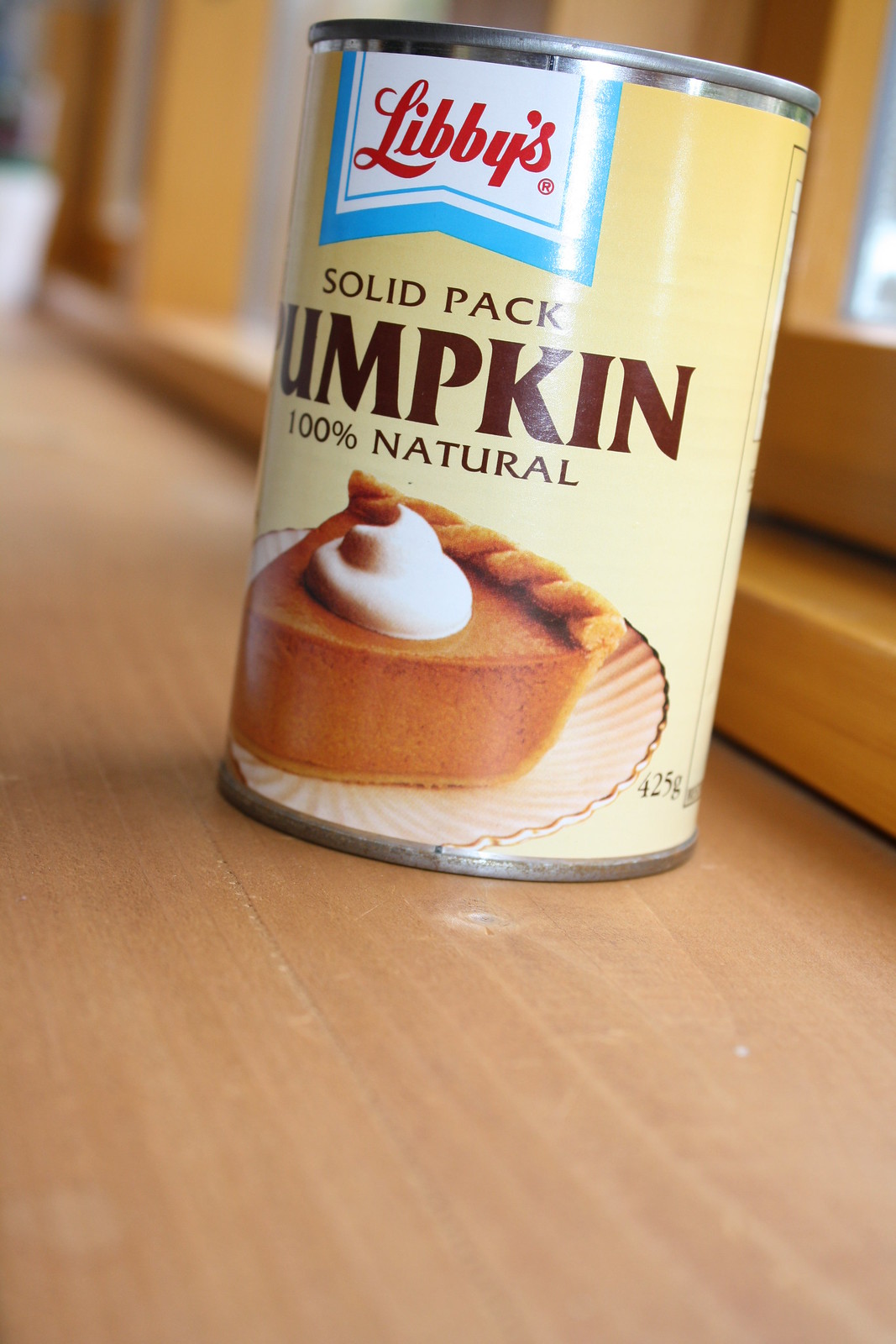This detailed photograph captures the main focus of a can of pumpkin, prominently placed in a kitchen setting. A slightly blurry background reveals a wooden windowsill with an orange-brown hue, where the can rests atop a light wood grain tabletop or counter. The can, cylindrical and topped with a silver lid, features a light brown label that fades to off-white. Dominating the top portion of the label is a rectangular area, outlined in light blue with a white background and the red text "Libby's." Central to the label, in dark brown letters, are the words "solid pack pumpkin 100% natural." At the bottom of the label, an appetizing slice of pumpkin pie adorned with a dollop of whipped cream is shown on a white plate with a gold rim. The detailed graphic reinforces the product's usage, making the can an inviting and central element of the image.